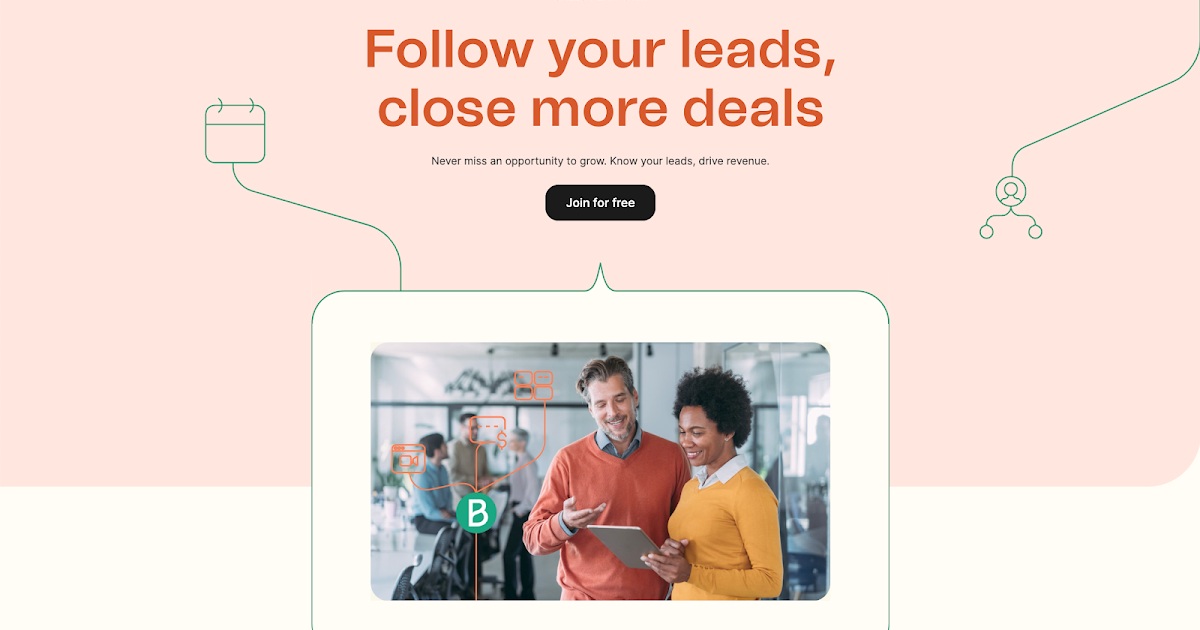The image, taken from a website with a light pink background, features a prominent message at the top in a reddish-orange font that reads, "Follow your leads, close more deals." Below this, in black print, it says, "Never miss an opportunity to grow. Know your leads, drive revenue." Centrally placed on the image is a clickable black button with white text that says, "Join for free."

In the foreground, there is a picture of a man and a woman. The woman is wearing a yellow shirt with a white collar and is holding a tablet or notebook. The man, dressed in an orange shirt with a gray collar, is smiling and pointing or gesturing as if to direct her attention to something specific. 

Beside them is a green circle with a capital letter 'B' in white inside it. Radiating from the circle are several orange lines suggesting connectivity. Surrounding these lines are various icons, including a video camera, a dollar sign, and four small boxes, with green lines symbolizing connections branching out and upwards.